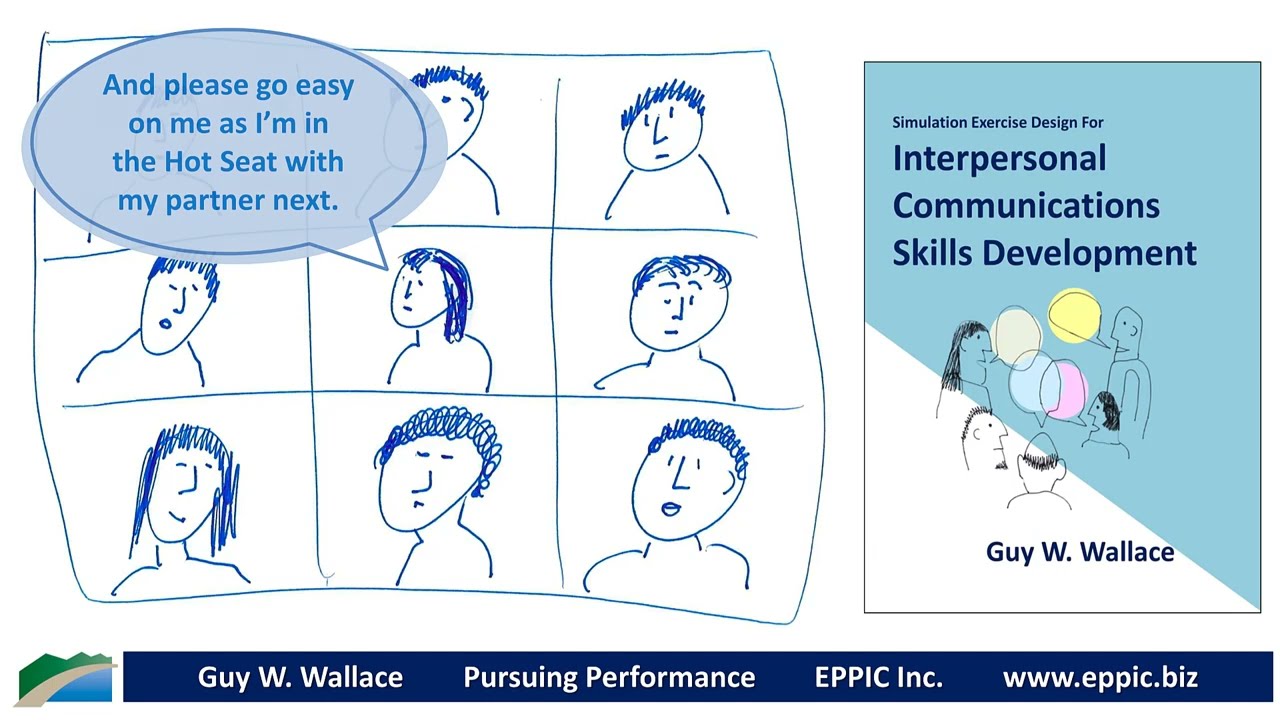The image resembles a professional presentation slide designed for adults, with a blue and white theme. On the right side, there is a rectangular visual element that looks like a book cover or pamphlet titled "Simulation Exercise Design for Interpersonal Communication Skills Development" by Guy W. Wallace. Below this title, in a blue band at the bottom, the text "Guy W. Wallace, Pursuing Performance, Epic Inc.," along with the website "www.epic.biz" is displayed in white font.

To the left of this visual, there is an illustration of nine faces arranged in a 3x3 grid, reminiscent of "The Brady Bunch" style. These faces are simple, sketch-like drawings. The central face in the grid features a speech bubble with the text, "And please go easy on me as I'm in the hot seat with my partner next." The overall design is detailed and structured to facilitate the development of interpersonal communication skills.